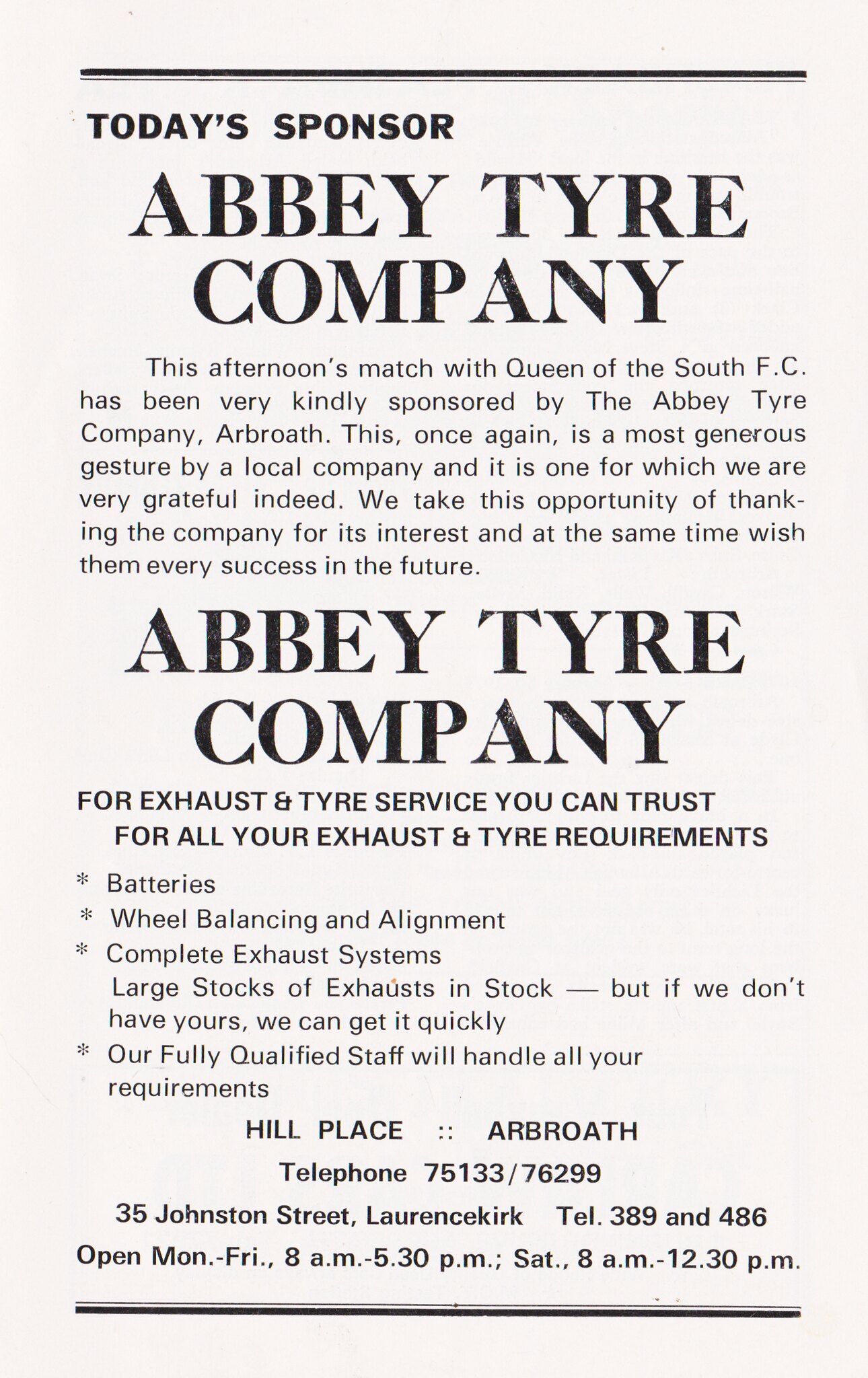**Abbey Tire Company Advertisement**

This full-page advertisement, likely placed inside a bulletin or program, prominently features today's sponsor, Abbey Tire Company. The layout is predominantly in black and white, topped with a horizontal black line. Below this line, "Today's Sponsor" is written in bold letters, followed by "Abbey Tire Company" in larger, prominent black letters.

A well-written paragraph highlights Abbey Tire Company's sponsorship of this afternoon’s match with Queen of the South FC, describing it as a generous gesture by a local firm. The community’s gratitude and best wishes for the company’s continued success are expressed warmly.

Continuing, the advertisement emphasizes Abbey Tire Company’s services with the repeated headline, "Abbey Tire Company." Beneath it, a subtitle reads, "For exhaust and tire service you can trust for all your exhaust and tire requirements." A comprehensive list details vital car maintenance services, crucial during the era of early automobiles, including batteries, wheel balancing and alignment, and complete exhaust systems. Special attention is given to their large stock of exhausts, with a promise of quick procurement if a specific item isn't available. The ad highlights the expertise of the fully qualified staff handling all customer requirements.

Contact information, including telephone numbers and addresses, is provided, and the page is neatly bordered with another horizontal black line at the bottom, framing the advertisement with precision. 

The historical context, the services offered, and the company's strong community ties are intricately detailed, presenting Abbey Tire Company as a reliable and essential service provider for early automobile enthusiasts.